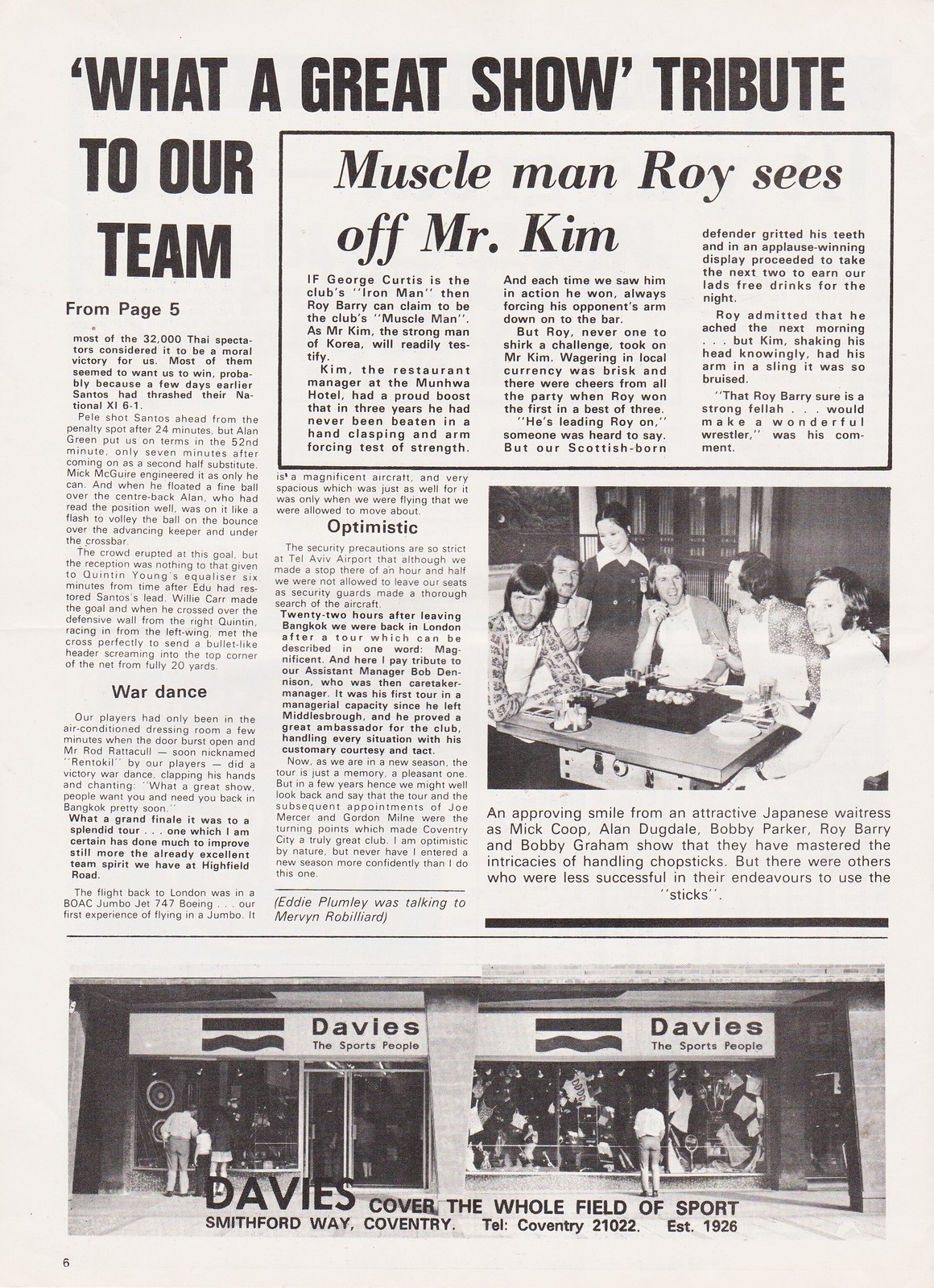This detailed newspaper clipping, titled "What a Great Show: Tribute to Our Team," features an article about an impressive demonstration of strength and camaraderie. The main headline captures the story's essence: "Muscle Man Roy Sees Off Mr. Kim." It chronicles Roy Berry's triumph over Mr. Kim, the renowned strongman and restaurant manager at the Manhwa Hotel, who had an unbeaten record in a hand-clasping and arm-forcing test of strength for three years. The article describes how wagering was brisk, with cheers erupting from the party when Roy won the first in a best-of-three challenge, ultimately leading to his victory. 

The newspaper clipping includes a black and white, old-timey photograph showing a group of men seated at a table, presumably celebrating. An approving smile from an attractive Japanese waitress in the background highlights the convivial atmosphere, as the diners handle chopsticks with varying degrees of success. At the bottom of the page, there is an advertisement for a sports store, "Davies," which proudly claims to cover the whole field of sports. The ad includes the store's address, "Smith-Firdway, Coventry," and a telephone number, "Coventry 21022."